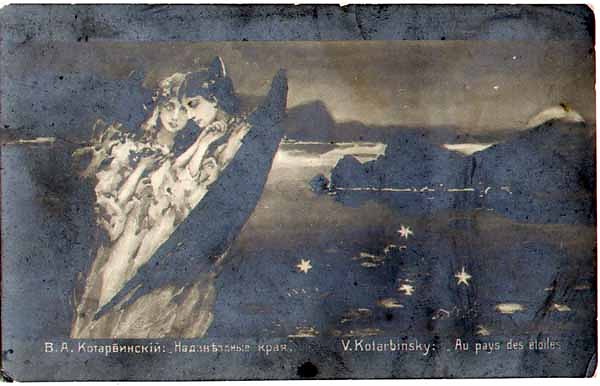The image is a detailed and atmospheric painting or possibly an early monochrome print by a Russian artist named V. Kolarbinsky. The artwork features two women, potentially angelic figures with long, dark hair, depicted on the left side. They are wearing flowing white dresses, and one appears to have wings. One woman has her hands near her chin, gazing downward, while the other looks forward with her hand across her chest. They are standing in a dark, abstract landscape featuring a gray sea or pond dotted with star-like flowers resembling lotus blossoms. Jagged rocks jut up through the water, and the backdrop is filled with faded mountains under a dim, blue-toned sky. Text at the bottom of the image, written in Russian, includes the names "R.A. Kopanecki" and "V. Kolarbinsky." The scene has a mysterious and almost ethereal quality, enhanced by the monochromatic color palette.